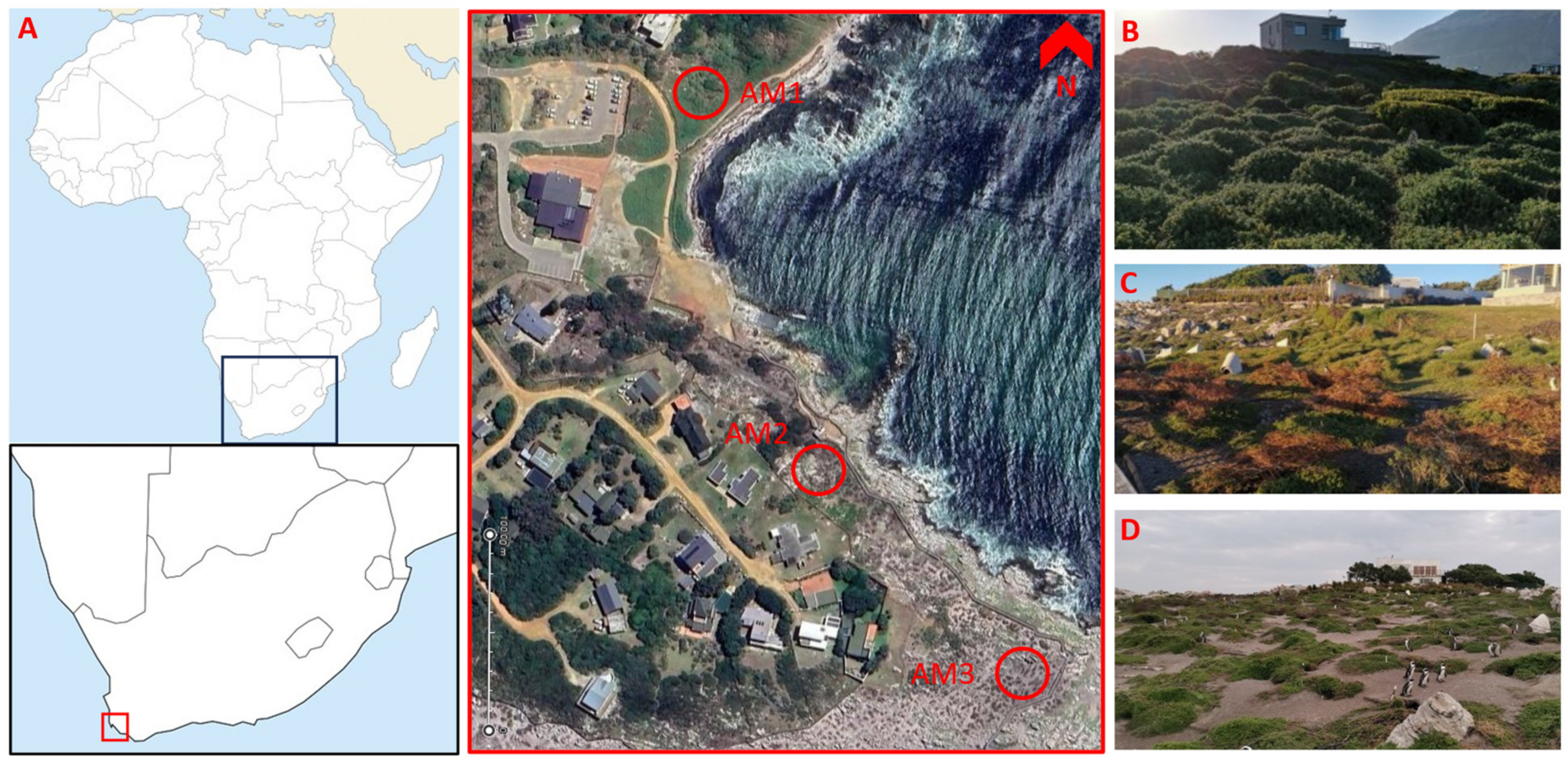This composite image provides detailed geographic and landscape information about the southern tip of Africa. The leftmost portion features a large, basic map of the African continent with a highlighted box indicating the focus area at the continent's southern tip. Below this is an enlarged section showing the Cape of Africa, marked with a smaller red square. The central image is a satellite or aerial photograph focusing on this smaller red-squared area, depicting water bodies, coastal regions, buildings, and roads, annotated with red markings, circles, and letters for further clarity.

To the right are three ground-level photographs that capture different aspects of the landscape within the highlighted area. The topmost image showcases a hill dotted with numerous bushes and what appears to be a small house perched on top. The middle image features a flatter terrain with abundant greenery, stones, bushes, and some buildings in the background. The bottom image displays a mixture of sand and greenery, including scattered low-lying ground cover and some black and white birds, likely seabirds, walking around. In the background, one can also discern a building and trees at a distance, with white stones visible throughout the landscape. Overall, this montage offers a comprehensive visual representation of the varied terrain and human habitation at Africa's southernmost point.